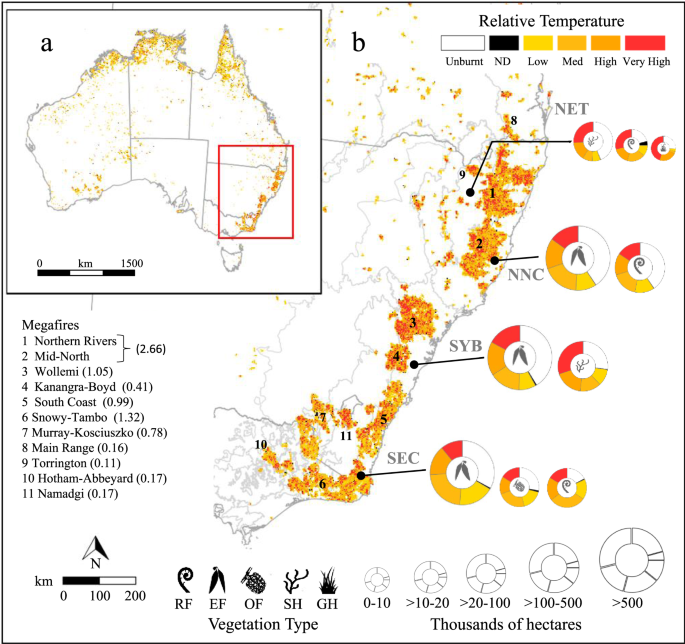The image is an intricate geographic map focused on the megafires in Australia. In the top left, there is an overview map of Australia with a red square indicating the zoomed-in region displayed on the right side. This larger section, labeled as part B, provides detailed insights into specific areas affected by fires. On the top right, a 'relative temperature' scale illustrates varying burn intensities: white for unburnt areas, black for ND (No Data), yellow for low intensity, light orange for medium, darker orange for high, and bright red for very high. The main map features a coastal region with different colored areas signifying temperature levels and small circles marking various types of vegetation as per a key at the bottom. This key uses pictures and acronyms to categorize vegetation types, also showing their sizes in hectares. Additionally, on the left side, there is a scale indicating how many kilometers per inch or centimeter, alongside a list of ongoing megafires and their geographical impact. Lastly, a compass in the bottom left corner indicates the map's orientation, pointing north.